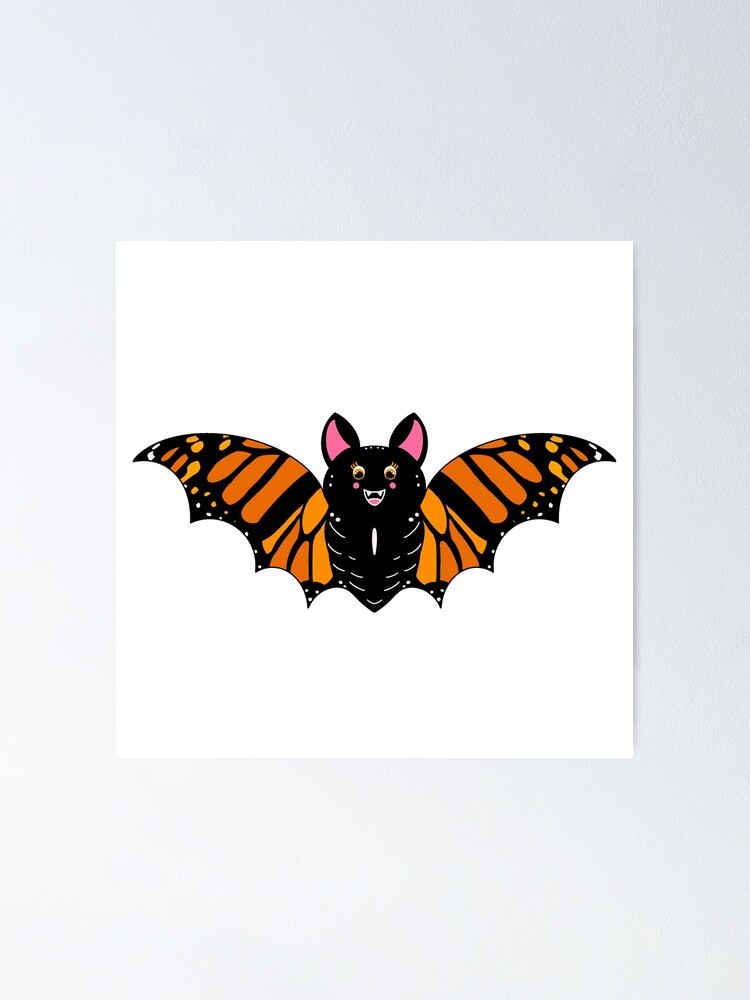This photograph depicts a square canvas hanging on a slightly less white wall. Central to the image is a whimsical cartoon bat rendered in a style reminiscent of a blend between a bat and a monarch butterfly. The bat features bright, decorative wings that extend left and right, adorned in shades of orange and black with hints of yellow, mirroring the intricate patterns of butterfly wings. The creature’s body and head are black, accented by a white slash on its breast. Its face is animated with yellow eyes that have black pupils, pink ears with black edges, and a cheerful expression showcasing a pink mouth with two small white teeth. The bat also has round pink blush marks below its eyes and yellow eyelashes, suggesting a feminine touch. The overall aesthetic makes this image feel computer-generated, aimed at a light-hearted or child-friendly audience.